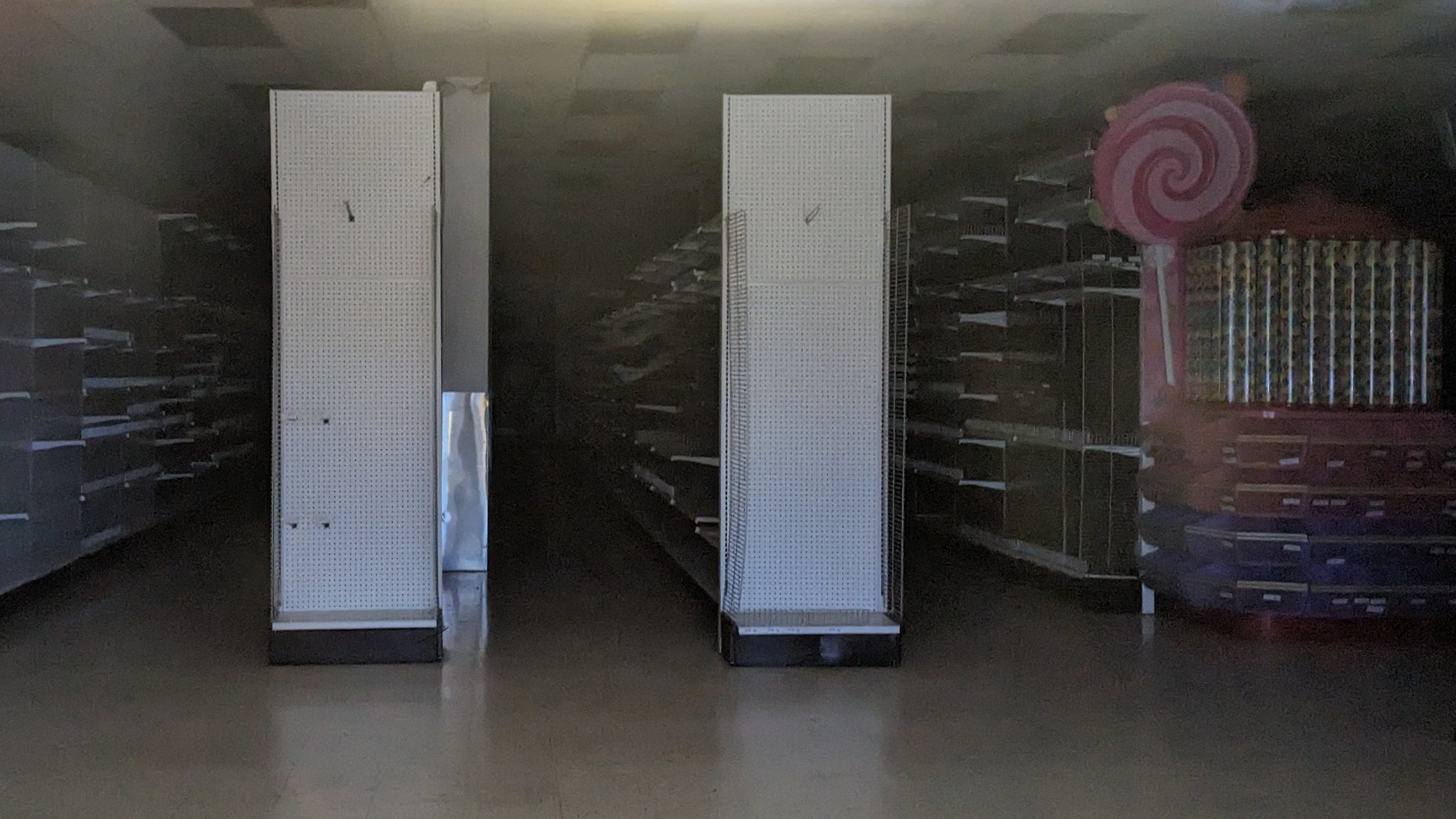The photo captures a dimly lit warehouse, emphasizing its stark and expansive interior. Dominating the scene are four prominent rows of metal shelving, perfectly aligned and extending into the shadowy depths of the warehouse. In the upper right corner of the image, one of the shelving rows culminates in a large pallet stacked with oversized plastic containers filled with colorful candy. This display is conspicuously accented with a large, round, pink swirled lollipop, positioned prominently on its left side, adding a whimsical contrast to the industrial setting. The ceiling, clearly visible in the shot, is composed of white tiles interspersed with dormant fluorescent light fixtures. The overall atmosphere is further accentuated by the cold, unyielding concrete floor that stretches across the warehouse.